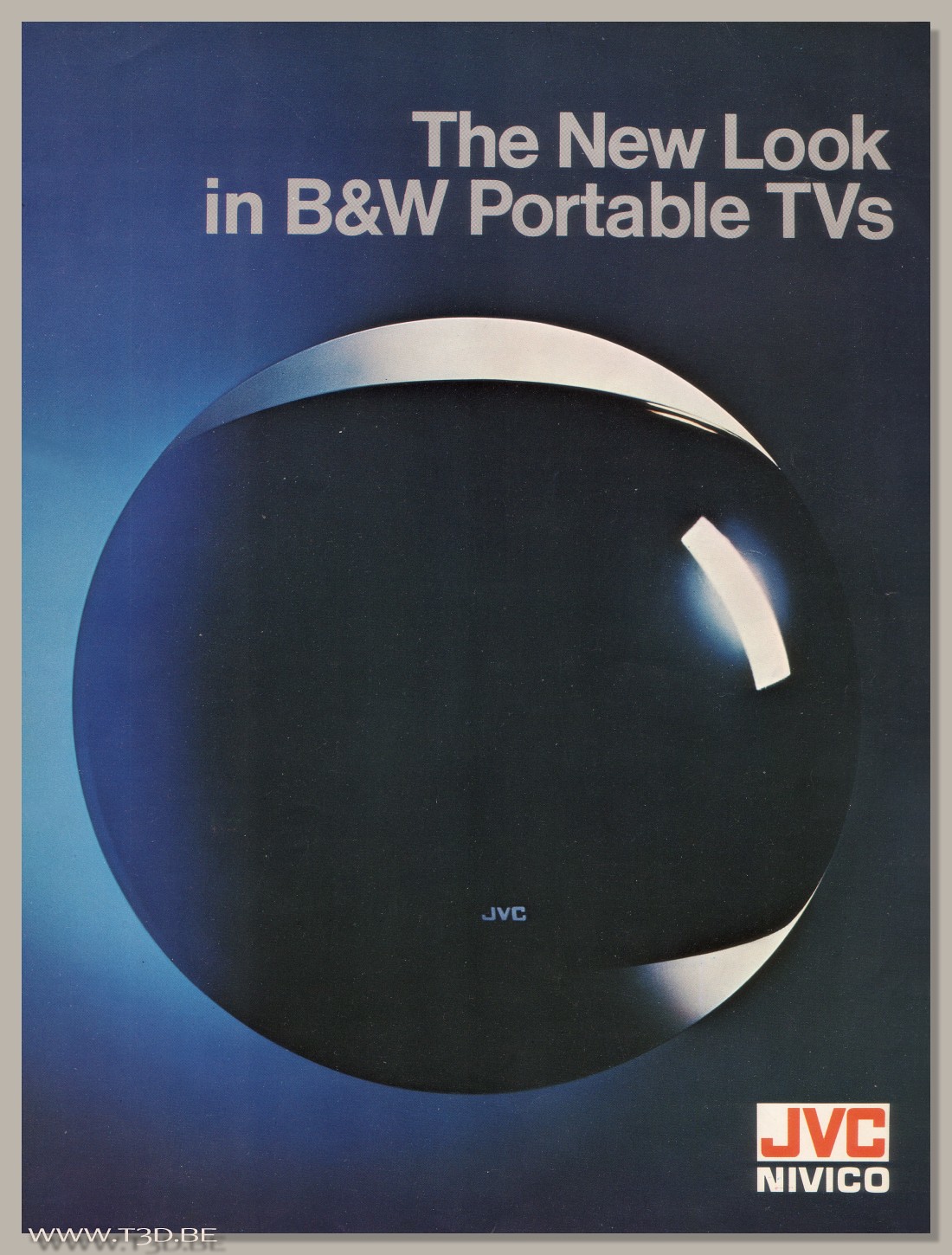This advertisement for JVC is set against a backdrop that transitions from dark blue to light blue, with the darker hues primarily at the top and the right-hand side. At the top right of the image, gray text announces, "The new look in B&W portable TVs." Dominating the center of the image is a large, spherical object resembling a marble, featuring a gradient from white at the top to black in the middle, with shades of gray and light blue towards the bottom left. The letters "JVC" are subtly positioned near the bottom of the sphere. In the bottom right corner, "JVC" is displayed prominently in red letters inside a white box, with "NIVICO" written below. Additionally, the website www.t3d.be is discreetly noted in the bottom left corner. This suggests a sleek, possibly innovative design for a portable TV by JVC, hinted to be either round or spherical in form.